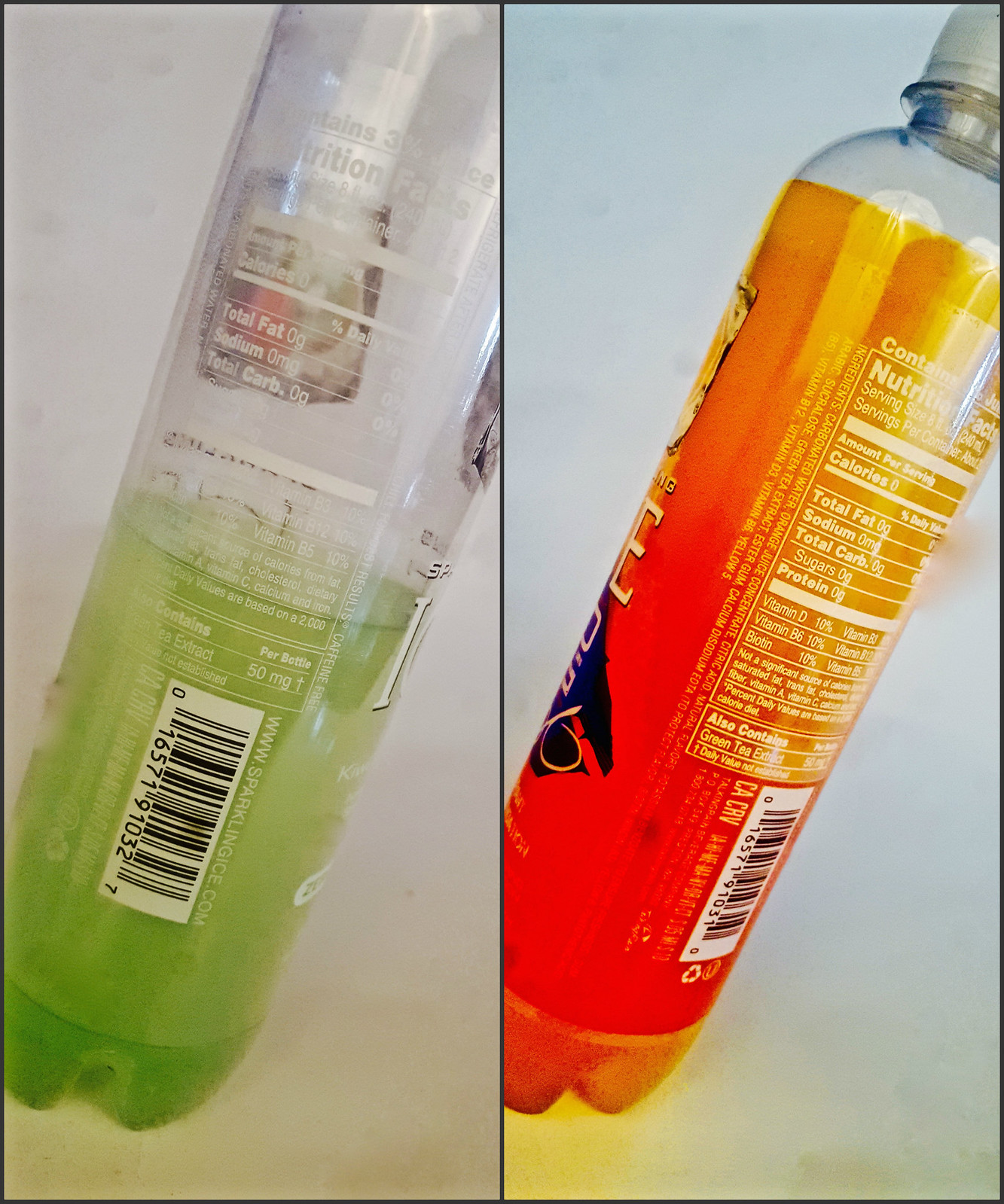This image features two bottles of sparkling ice drinks positioned side-by-side against a plain background. The bottle on the left is a half-empty, transparent green bottle. Though it's difficult to discern all the details, you can see parts of the nutrition label and barcode clearly displayed on its back. Notably, the label mentions "Green Tea Extract, 50 milligrams per bottle." Due to the bottle's transparency and its partially consumed content, the top half appears empty, making the liquid level distinctly visible. The bottle on the right, corresponding to the left side from the viewer’s perspective, is an unopened orange-flavored sparkling ice drink. The front of this bottle reveals a partial view of the letter 'E' and a small segment of the design, hinting at its branding. The back also shows a nutrition label with difficult-to-read details listing calories, total fat, sodium, total carbohydrates, sugars, protein, vitamin D, vitamin B, and biotin, along with green tea extract content. A barcode is present at the bottom. Overall, both bottles are positioned to reveal nutritional data and barcodes despite the partial obstruction of some details.